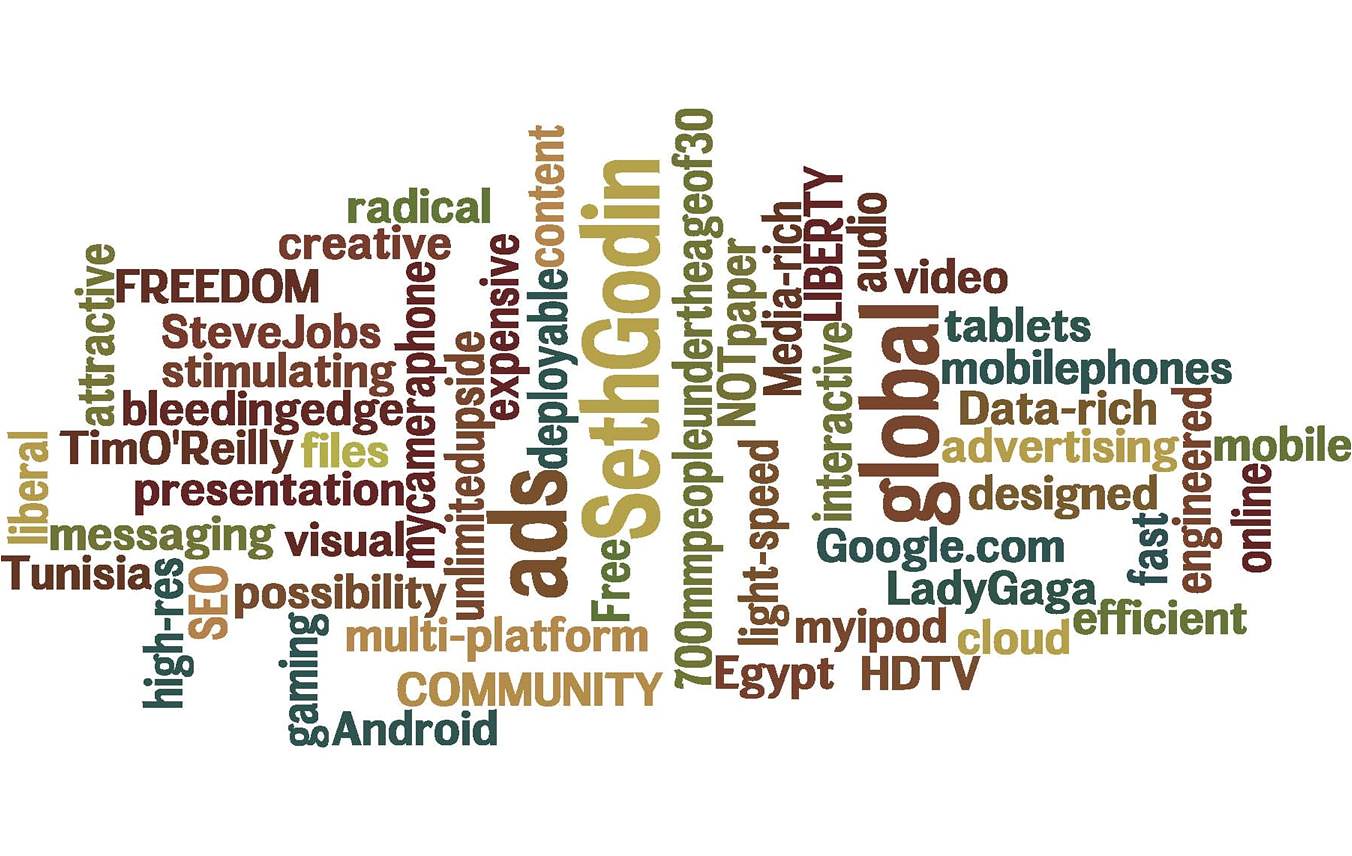The image portrays a detailed word cloud with a variety of seemingly random names and terms, presented in numerous colors and sizes, illustrating a broad array of themes. The largest and most prominent words in the cloud include "Seth Godin" in a yellowish-brown hue, "global" in brown, and "ads" also in brown. Arranged both horizontally and vertically, the words cover different aspects such as technology, freedom, and media, depicted in shades of brown, green, blue, and a muted beige.

Noteworthy mentions encompassing both popular figures and concepts include "Steve Jobs," "Tim O'Reilly," "Lady Gaga," "android," "liberty," "presentation," "freedom," and "mobile phones." The left side of the cloud features horizontal words like "freedom" in brown, "radical" in green, "creative," and "multi-platform" in maroon, while the right side includes "video," "tablets," "advertising," and "google.com."

Vertical words occupy the center and outer edges, with "Seth Godin" standing as the largest. Other significant vertical entries include "not paper," "interactive," and "engineered." Lesser emphasized but still notable terms include, "liberal," "attractive," "stimulating," "bleeding edge," "Tunisia," "hi-res gaming," "deployable," and "efficient." The words "free" in vibrant green and "data-rich" in blue add to the varied thematic presence within the word cloud. This intricate collage visually emphasizes marketing, technology, and modern digital experiences through its diverse lexicon.